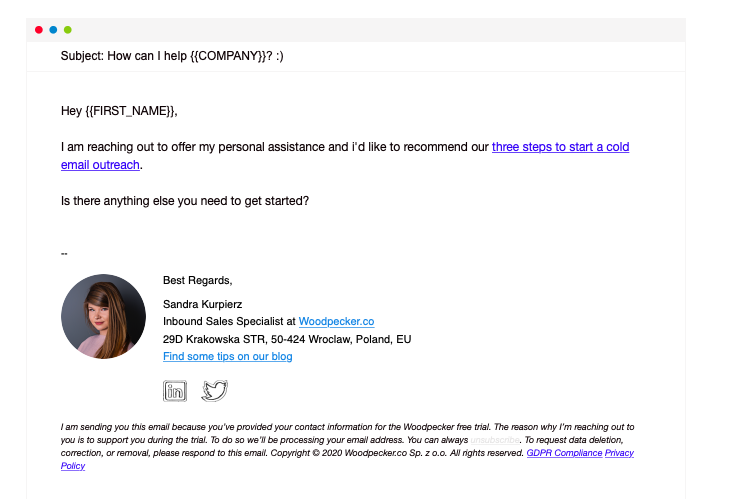This image depicts an email template designed to resemble the Mac OS interface, evident from the UI elements positioned at the header. The background of the email is white, enhancing its minimalist design.

At the top, there’s a section labeled "Subject," which reads "How can I help," followed by a placeholder variable {{COMPANY}} in uppercase and enclosed by double brackets. This suggests that the template employs variables, similar to programming placeholders.

The body of the email begins with a greeting, "Hey {{FIRST_NAME}}," again, with the recipient's first name functioning as a variable. The email continues with a personalized offer: "I am reaching out to offer my personal assistance and I'd like to recommend our three steps to start a cold email outreach." The phrase "three steps to start a cold email outreach" is highlighted with a blue underline, indicating it is a clickable link.

The following sentence asks, "Is there anything else you need to get started?" Below this, the signature section includes a photograph of the sender, who appears to be of European descent, with light peachy skin and long brown hair. To the right of the photograph, it reads:

"Best regards,  
Sandra Kurpiers,  
Inbound Sales Specialist at Woodpecker.co,  
29D Krakowska Street, Poland."

Underneath this, there is a link with the anchor text "Find some tips on our blog," which directs to additional resources. Following this are icons for LinkedIn and Twitter, leading to the social media profiles of the company. The footer concludes with copyright information and other necessary legal statements.

Overall, the email template is professionally structured to incorporate dynamic content, links to resources, and convenient access to social media, making it a versatile tool for outreach efforts.